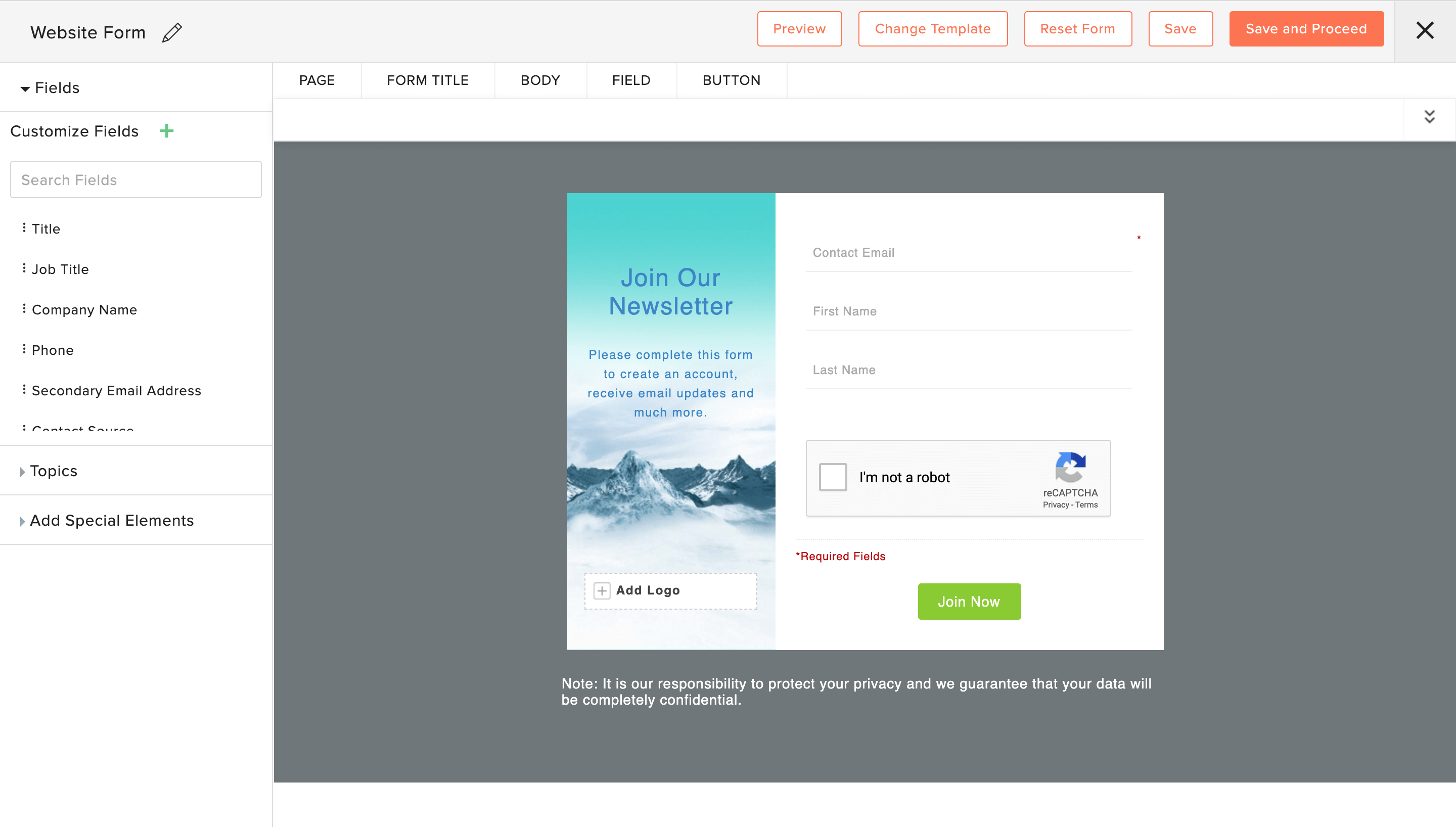**Detailed Caption:**

This image is a screenshot of a website form customization interface. At the top left corner, there's a label that reads "Website Form" accompanied by a pencil icon, signifying editability. To the right of this bar, there are several functional buttons in sequence: "Preview," "Change Template," "Reset Form," "Save," and "Save and Proceed." These buttons are styled with a white background, orange outlines, and orange text, except for the "Save and Proceed" button, which is orange with white text. An "X" icon is situated to the far right, likely for closing the interface.

Below the top bar, there is a form layout. The left side features a headline, "Join Our Newsletter," followed by a description: "Please complete this form to create an account, receive email updates, and much more." Underneath this text is an image depicting mountains, adding visual interest to the form.

On the right side of the form, there is a contact form section with fields labeled "Contact Email," "First Name," and "Last Name." A CAPTCHA verification component is located below these input fields, ensuring user authenticity. The design and layout emphasize functionality while maintaining a clean and user-friendly aesthetic.